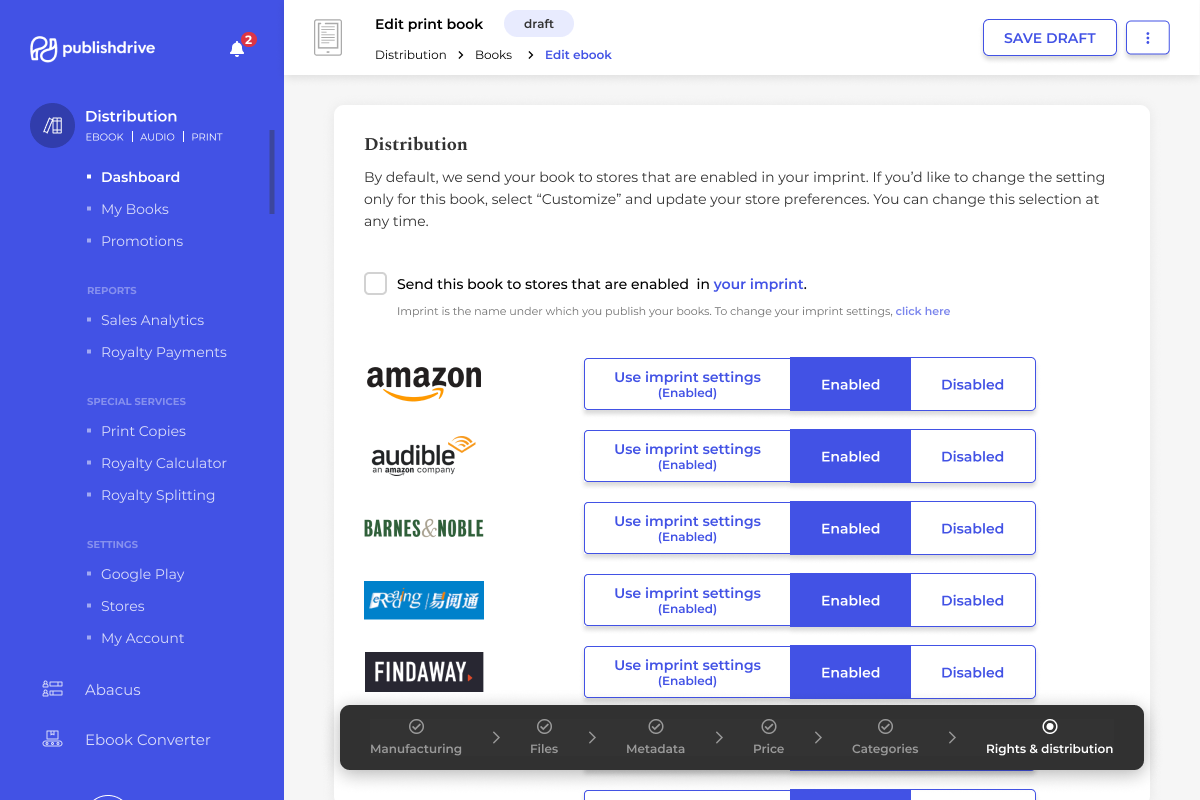Here is a cleaned-up and detailed caption based on the provided description:

---

A detailed desktop screenshot showcasing the PublishDrive interface, set against a predominantly blue background. In the top left corner, the PublishDrive logo incorporates a yin-yang-esque design resembling inverted Apple AirPods. Adjacent to the logo on the right, a notification bell icon displays the number '2', indicating two pending notifications. Below, the main menu features tabs for "E-book," "Audio," and "Print," currently on the "Distribution" tab.

Beneath these tabs, the sidebar menu lists several key sections:
1. **Dashboard** (highlighted)
2. **My Books**
3. **Promotions**

Followed by headers and their corresponding bullet points:
- **Reports**
  - Sales Analytics
  - Royalty Payments
- **Special Services**
  - Print Copies
  - Royalty Calculator
  - Royalty Splitting
- **Settings**
  - Google Play
  - Stores
  - My Account

Additional headers include "Abacus" and "E-book Converter."

In the top right corner, there is a rectangular "Save Draft" button and a square settings button with three vertically-aligned dots. Along the middle left portion of the screen, there is an "Edit Print Book" section. To its right, another draft button is visible, with navigation links below: "Distribution," "Books," and "Edit E-book." The "Edit E-book" link is highlighted in blue, confirming that the user is currently in the "Edit Print Book" interface.